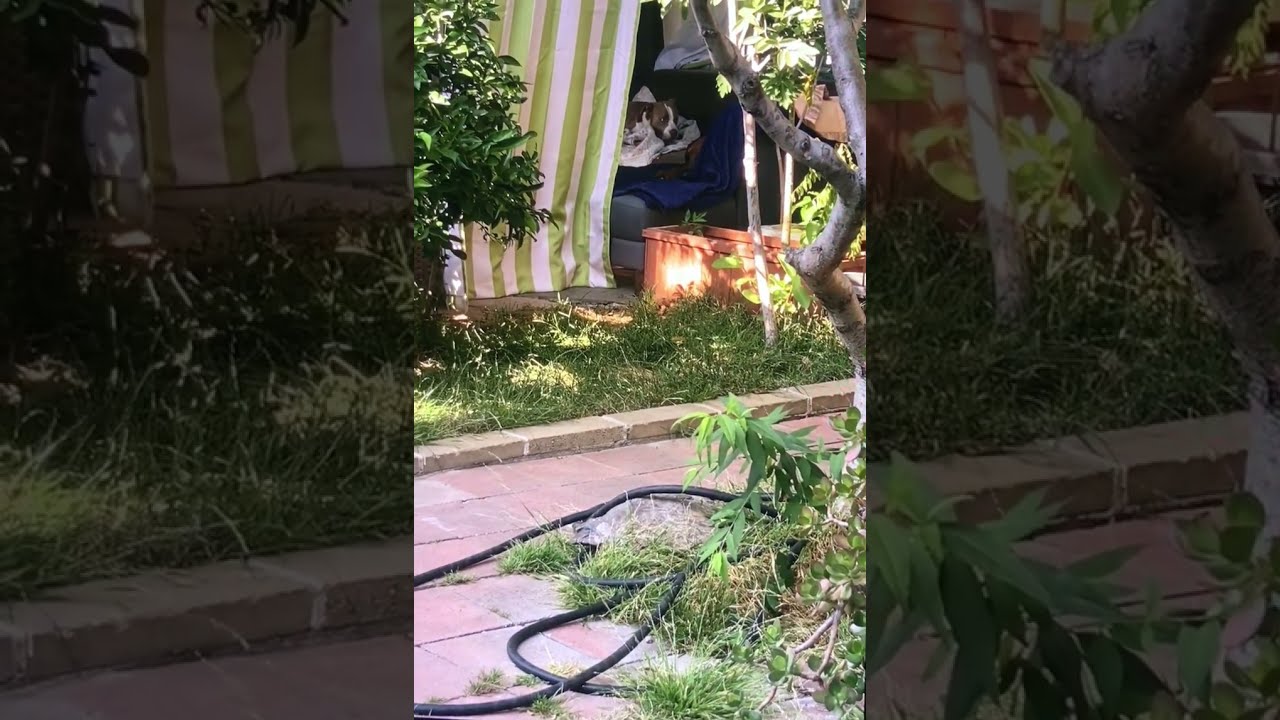The image depicts an outdoor setting, likely a backyard, featuring a variety of elements. At the bottom of the image, there's a brick-style tile patio with a large, black hose coiled and strewn across it. Adjacent to the patio, patches of grass and untrimmed bushes surround a thin-branched tree on the right side. The scene extends to the top of the image, which prominently features a gazebo or tent-like structure with green, lime green, and white striped awning. Inside this gazebo, there's a gray couch adorned with a blue blanket and a dog bed. A brown Boxer dog with a white stripe down its face rests comfortably on this dog bed. The overall setting is outdoors during daylight, filled with varying shades of green from the unkempt grass and foliage, and appears to be a relaxed, lounging area, possibly intended for capturing the dog's peaceful repose.